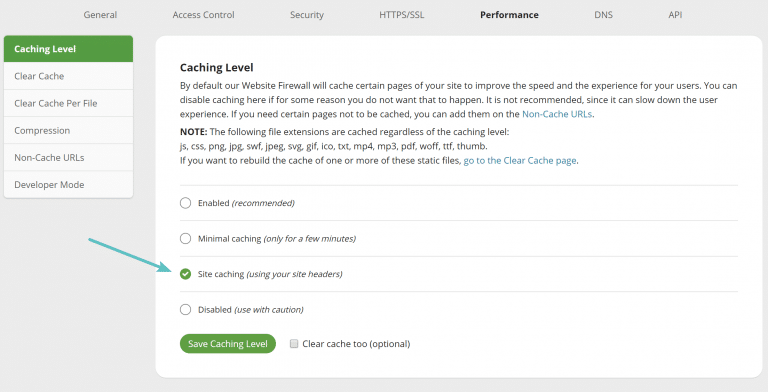The image displays a menu interface typically seen on a computer or mobile device. The main focus is a menu titled "Caching Level," which is prominently highlighted in green. On the left side of the screen, there's a vertical menu bar listing several options: Caching Level, Clear Cache, Clear Cache Profile, Compression, Non-Cache URLs, and Developer Mode. The "Caching Level" option is currently selected, drawing attention to an expanded informational window on the right side of the screen.

This expanded window provides a thorough explanation of what the "Caching Level" feature entails. Below the general information, there are four selectable options related to caching strategies. Among these, the option "Site caching using your site headers" is currently chosen.

At the bottom of the window, there is a pair of interactive buttons. The first one, highlighted in green, reads "Save Caching Level," allowing users to save their settings. Adjacent to it is an alternative button labeled "Clear Caching Level," offering the option to reset the settings.